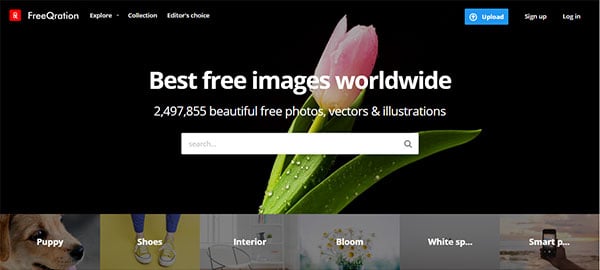The top section of the image features a red square with the text "Free Curation" and options like "Explore," "Drop Down Menu," "Collection," and "Editor's Choice." On the far right, there is a rectangular area with buttons for "Upload," "Sign Up," and "Log In."

In the center of the image, prominently displayed, is the phrase "Best Free Images Worldwide." Beneath this, there is a background of green leaves and pink flowers. Below the background, a text reads "2,497,855 beautiful free photos, vectors, illustrations." 

Underneath this text, there is a search bar. Next, an area displays various tag thumbnails: 

- A brown puppy, centered with the text "puppy," appears repeatedly.
- Yellow shoes and blue interior images are also depicted.
- Further to the right, an assortment of flowers against a white square backdrop with text that reads "Smart" and mentions something resembling a phone, indicating an assortment of stock photos.

Overall, the image presents an extensive collection of free, high-quality photos, vectors, and illustrations, emphasizing easy exploration and user interaction options such as uploading, signing up, and logging in.